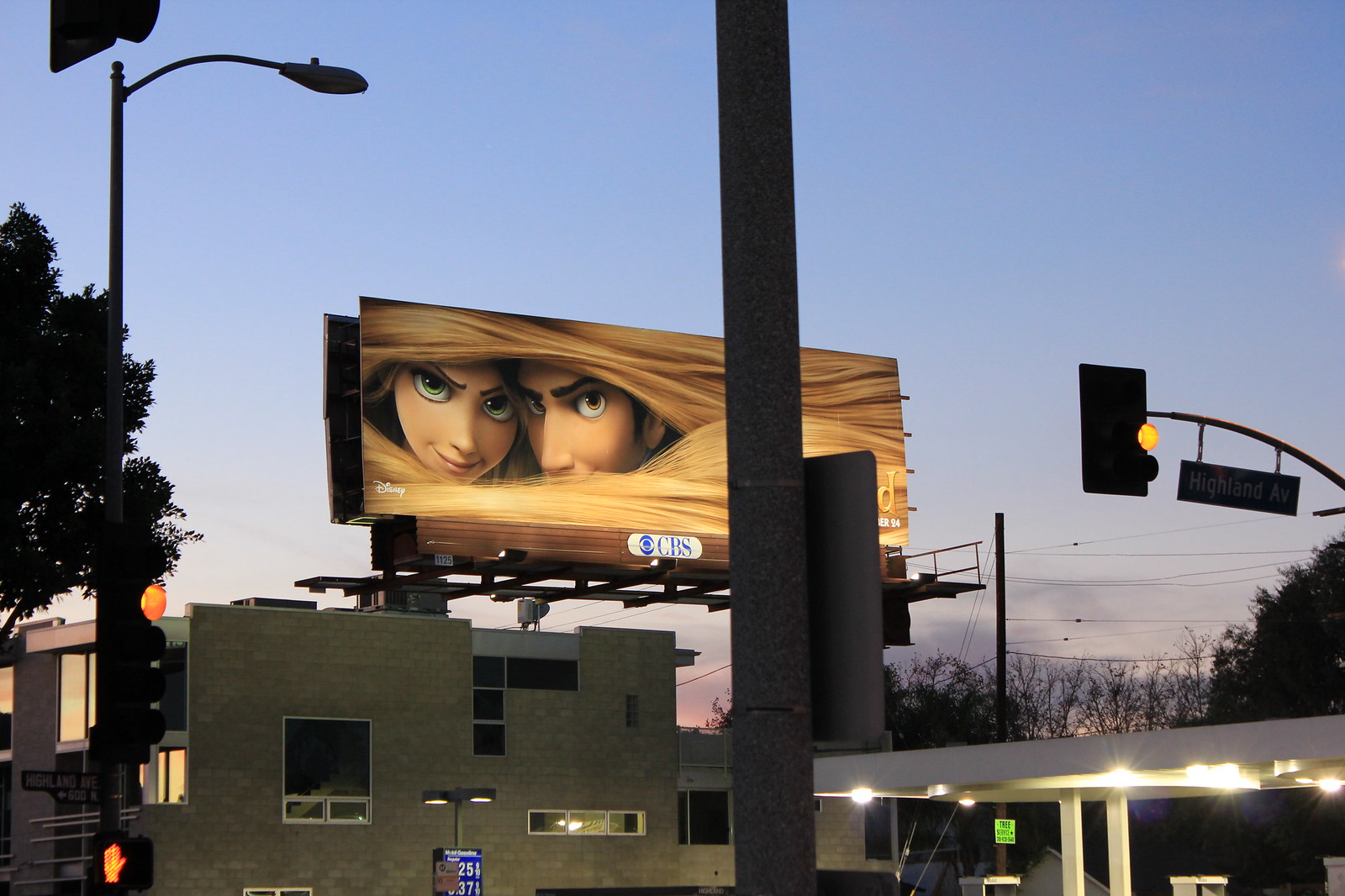This photograph captures a twilight scene featuring a vibrant billboard advertisement for the computer-generated movie "Tangled," a modern remake of the classic tale of Rapunzel. The billboard prominently displays Rapunzel and her love interest emerging from her extensive, golden hair, against a backdrop of a scenic landscape. Beneath the billboard, a distinctive building with gray brickwork and an eclectic array of windows adds an artsy touch to the scene. On the lower right, there's a gas station, marked by visible prices and the yellow glow of a traffic light transitioning, while in the distance, trees and electricity lines create a layered backdrop. The CBS logo is situated below the main advertisement on the billboard, reinforcing the connection to mainstream media. The distinct twilight ambiance captures the subtle hues of an impending sunset, casting a serene light over the entire scene.